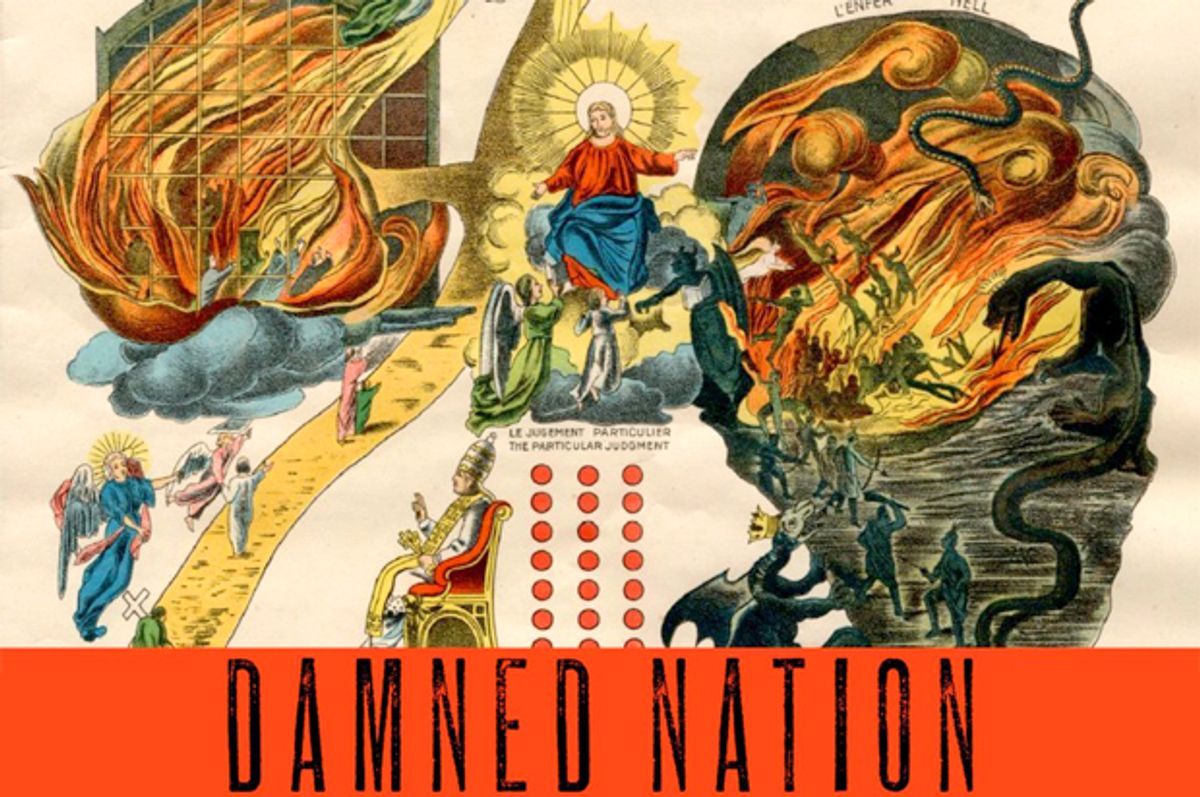In this intricate and vividly illustrated image, we have a detailed Christian-themed scene that is divided into contrasting realms of heaven and hell, with a gray-based background. Dominating the center of the illustration is a majestic figure, presumably God or Jesus, adorned in an orange robe with a halo, emanating divine light and authority. Surrounding him are kneeling angels in prayer, draped in red and blue garments. 

To the left-hand side of the image, a golden pathway lined with angelic figures extends, symbolizing the road to heaven. This path features various human characters, including one carrying a cross, moving along it towards a higher, divine purpose. The pathway connects to a heavenly realm filled with clouds and more angelic figures.

In stark contrast, the right-hand side of the image plunges into the chaotic vision of hell. This area is alive with fiery hues of orange, yellow, and red engulfing demonic figures, serpents, and dragons. One prominent serpent winds its way towards the top right corner, adding an element of menace and turmoil to the scene. Amongst the flames and smoke, demonic entities exhibit twisted forms, highlighting the stark opposition between the realms.

At the very bottom of the image, the words "DAMNED NATION" stand out in bold black text against an orange banner, cementing the theme of divine judgment and the stark contrast between salvation and damnation.